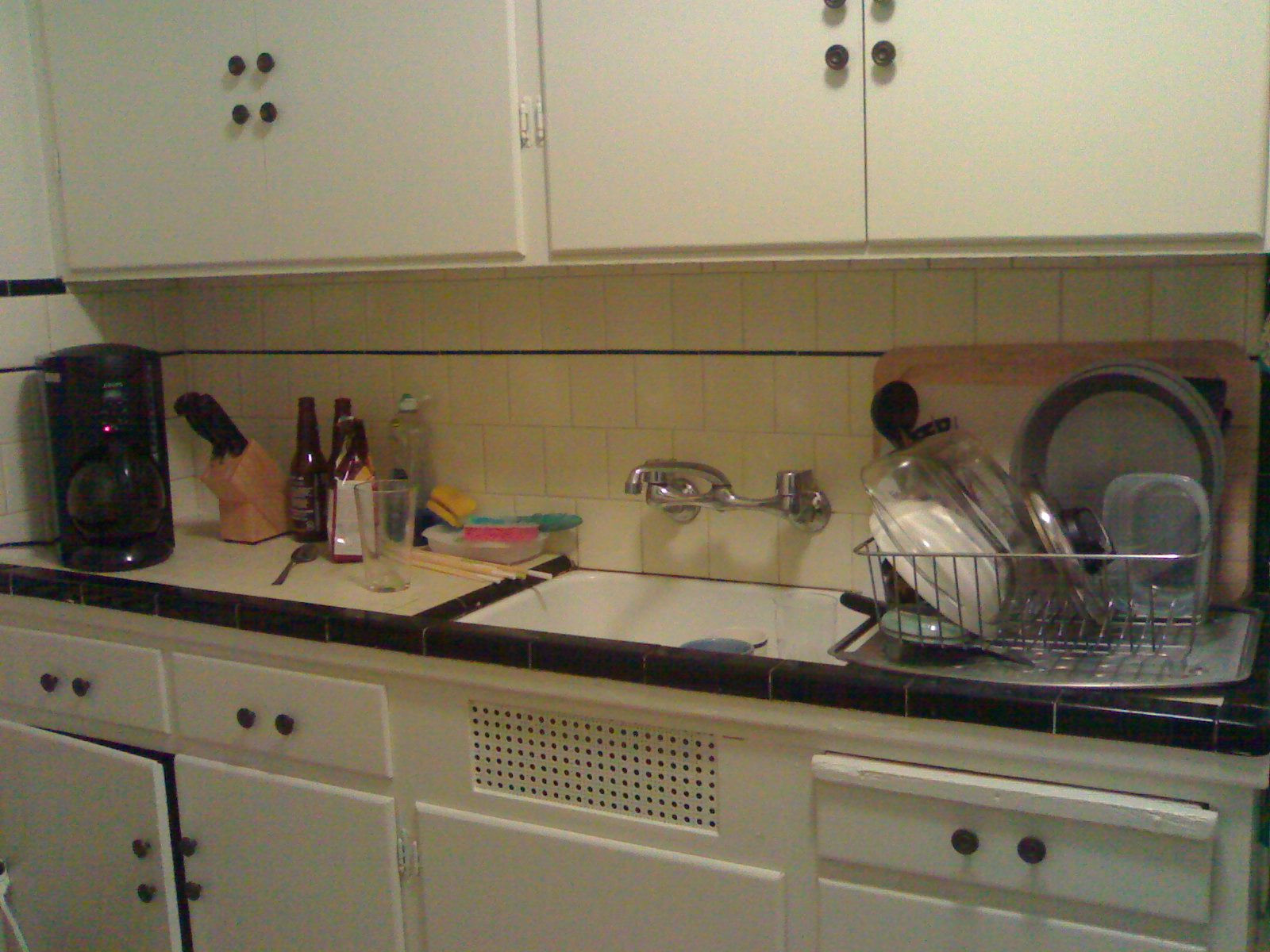In this image, the kitchen features sleek white cabinets at the top, each adorned with two small circular handles on either side, totaling eight circles. The cabinets are separated by a thin line. Below the cabinets, tan tiles form the backsplash, interspersed with a black line and more tan tile. 

On the left-hand side of the countertop, a coffee pot sits next to a knife holder filled with knives. Scattered nearby are various bottles, a spoon, a clear glass, and a bottle of dish soap. A few chopsticks and a clear container holding multi-colored sponges—yellow, pink, and bluish-green—are also present.

Central to the image is a white sink with an unidentified blue item inside it. Beside the sink, a green dish drainer holds several clean dishes. The counter is bordered by a thin line of black tiles, giving it a refined look.

Below the counter, there are white drawers and cabinets. Each drawer has two small handles. A particular cabinet beneath the sink is slightly ajar and features two handles per door. Below the sink, there's a rectangular panel filled with numerous small black dots. To the right, another drawer with two handles is visible, alongside the top of an adjacent cabinet.

This detailed setting reflects a well-organized and functional kitchen space.